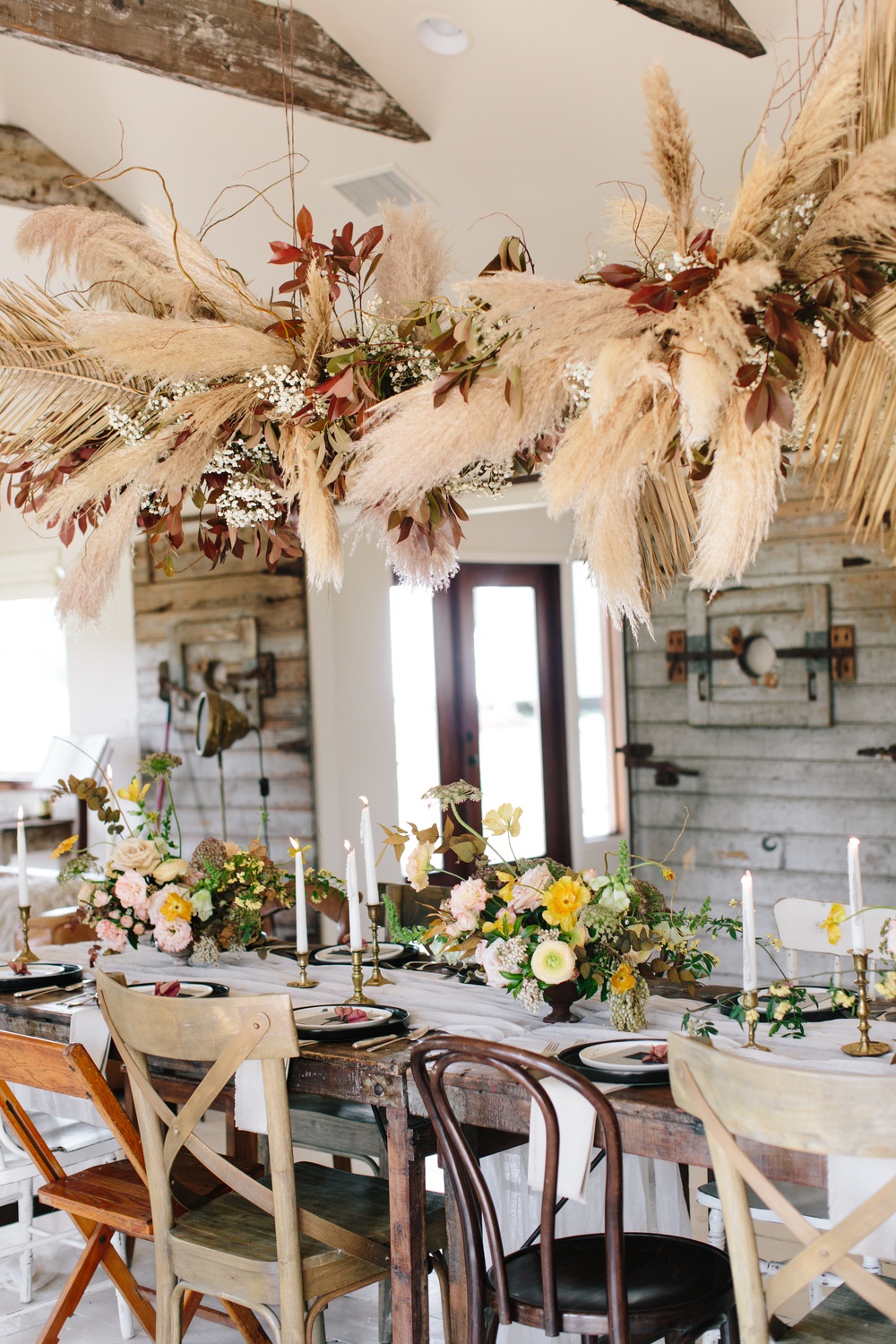The photograph captures a professionally staged, indoor setting of a dining area in a home. The focal point is a long, rectangular wooden table adorned with an array of different styled and colored wooden chairs. The table is elegantly set with brown-rimmed plates topped with white plates detailed with pink flowers, several gold candlesticks holding white candles, and multiple sophisticated flower arrangements featuring white, light purple, and yellow flowers along with green leaves. 

Above the table, hanging from the white ceiling supported by mostly brown wooden beams, is a striking decoration composed of fanned-out leaves, ferns, and darker flowers, adding a lush, natural element to the scene. Sunlight streams through a glass door with sidelights and a brown frame located centrally in the background. A side window enhances the indoor brightness, while a white brick wall adds texture to the backdrop. The visual harmony of the set-up is further complemented by a white tablecloth running down the middle of the table and a white sheet placed underneath it, contributing to the room's inviting and elegant atmosphere.